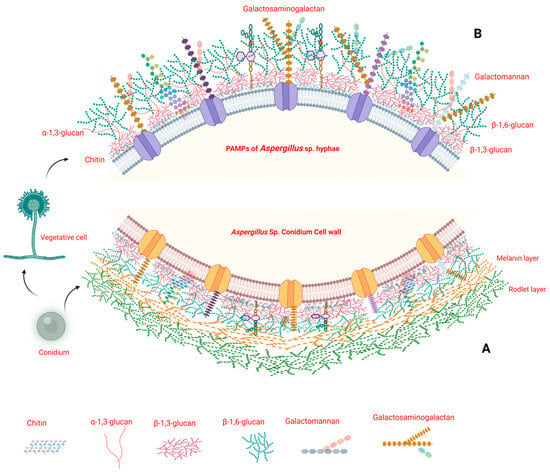This detailed image illustrates the deconstruction of a plant cell, specifically highlighting the cell wall components of Aspergillus species. Dominating the top of the image, the title "Galactosaminogalactan" is prominently displayed in red letters. The visual is filled with various colors and shapes, resembling tiny beads in shades of orange and purple, which are displayed in a pattern moving upwards.

Centrally, the image features two half-circle diagrams teeming with squiggles and scribbles, each dotted with five purple circles. Encircling these half-circles are varied hues transitioning from pink to yellow to green. The half-circles also contain captions indicating "PAMPS of Aspergillus hyphae" and "Aspergillus sp. Conidium cell wall," along with detailed molecular structures.

At the very bottom, a sequence of labeled images illustrates the structural components: chitin, 1,3-glucan, 1,3-glucan (again but possibly with different conformation), 1,6-glucan, galactomannan, and galactosaminogalactan. These elements are depicted as unique symbols, highlighting their distinct roles within the cell wall.

To the lower left corner, there is a small seed-like figure beside a green vegetative cell drawing, aligning with the caption "VEGETATIVE CELL" to the right of it. Overall, this image serves as a detailed scientific breakdown of the Aspergillus cell wall's composition and structure, showcasing its complex molecular diversity.